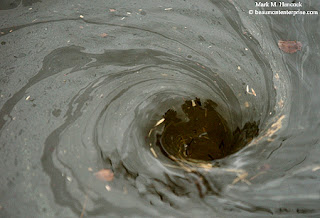This image is a close-up photograph depicting water swirling down a drain, creating a spiral pattern in a clockwise direction. The photograph, taken by Mark M. Thompson, includes a watermark in the top right-hand corner along with a copyright notice for a website, both of which are illegible. The scene captures murky, polluted water with various floating particles such as leaves and dirt, and possibly oil, giving the water a dark gray or brownish hue. The water appears to be draining into a hole, possibly on a street or another hard surface, emphasizing the motion of water being pulled down by the drain. The image is somewhat small and not in perfect focus, making it challenging to discern finer details.